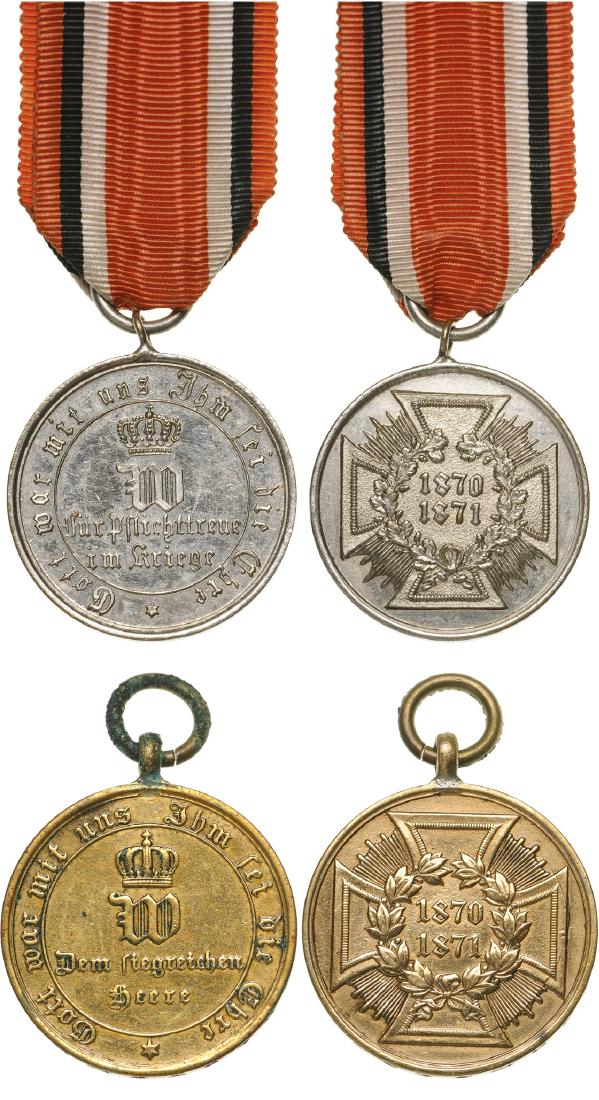This image showcases a set of four war medals, two silver and two gold. The top two medals are silver and are suspended from a ribbon that features black, white, and red lines. The medal on the left has a crown at the top with a letter "W" beneath it, encircled by non-English text along the edge. The right silver medal displays an iron cross with a wreath at its center, enclosing the years 1870 and 1871. Below these, the two gold medals replicate the design of the silver ones. The left gold medal mirrors the silver's crown and "W" design, while the right gold medal also features the iron cross with the same years, 1870 and 1871, inscribed at its center. Unlike the silver medals, the gold medals are unattached but have rings at the top, indicating they can be mounted or attached similarly.